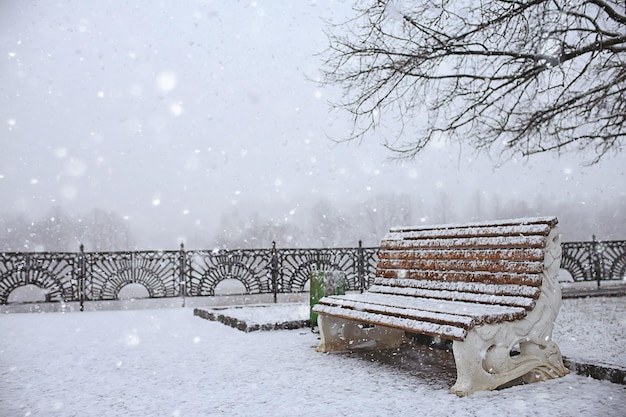In this serene image of a park blanketed in snowfall, a stone bench with wooden slats, now covered in snow, sits prominently in the foreground. The slats, slightly dusted with snow, suggest a recent and ongoing snowfall. Behind the bench, an ornate metal railing, designed with artistic sunburst or peacock feather-like patterns, adds a touch of elegance to the wintry scene. The railing, likely silver or black, contrasts beautifully with the white snow. To the right of the bench and in slight blur, a green trash can, also cloaked in snow, introduces a subtle burst of color against the predominantly monochrome backdrop. Dominating the scene further back are naked tree branches, stretching out like delicate fingers, devoid of leaves and standing stark against the gray sky. The sky itself carries a heavy blanket of clouds, with snow gently falling, adding layers to the pristine scene. The overall atmosphere is peaceful yet chilly, encapsulating the quiet beauty of a park in the midst of a snowfall.